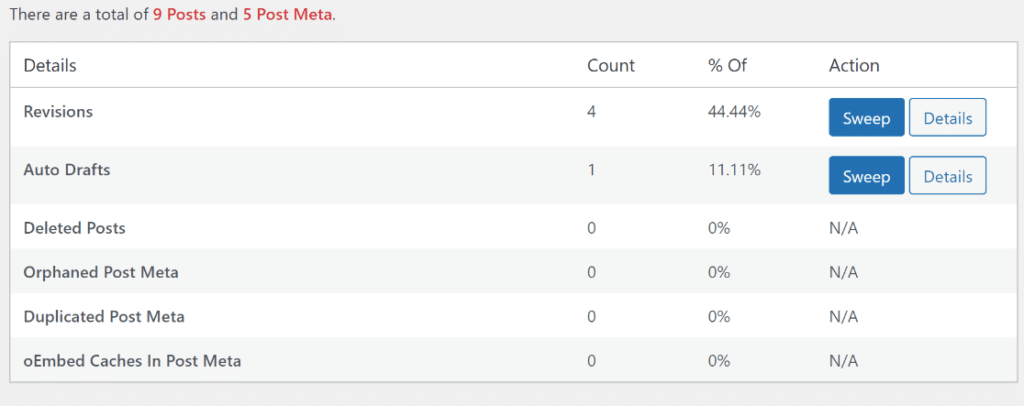**Descriptive Caption:**

This screenshot showcases an analytics page detailing various aspects of posts and their associated metadata. At the top section, the total number of posts and post meta are prominently displayed in red font—9 and 5 respectively—while the remaining text is in black. 

Directly below, the table is divided into four main headers: "Details," "Count," "Percentage Of," and "Action." The table contains six rows, each representing a different category: 
1. Revisions
2. Autodrafts
3. Deleted Posts 
4. Orphaned Post Meta
5. Duplicated Post Meta
6. Embed Caches in Post Meta 

In the "Count" column, the numbers 4, 1, 0, 0, 0, 0 are displayed corresponding to the categories listed. The "Percentage Of" column indicates that revisions account for 44.44%, autodrafts for 11.11%, with the remaining categories all showing 0%.

For the "Action" column, each row mentions specific options: "Sweep" and "Details" buttons are available for both revisions and autodrafts, whereas the other categories display "N/A."

Overall, this page provides a detailed analysis of the types and activities concerning different posts and their metadata, along with actionable options for further management.